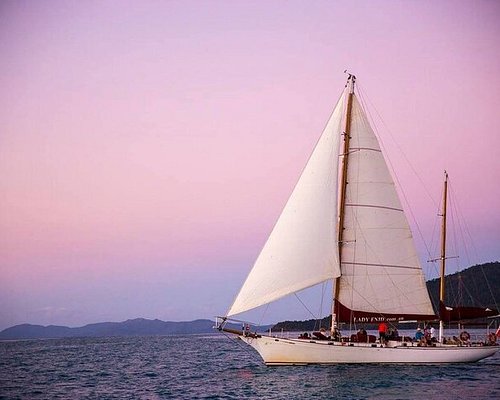In this computer-generated image, a white sailboat occupies the right side, with its bow pointing to the left and the stern to the right. The sailboat features two white sails and a brown mast and has a distinctive front area for observation. There are several people onboard, one wearing a red shirt, and the boat is equipped with a couple of life preservers. The boat bears the name "Lady Something," and the water around it appears slightly choppy, extending out of the frame at the bottom and right edges. The background showcases a picturesque landscape with hills on both sides. The sky presents an artistic blend of colors, transitioning from a light blue near the horizon to a purplish hue, with lavender tones at the top, creating a surreal and classy atmosphere.